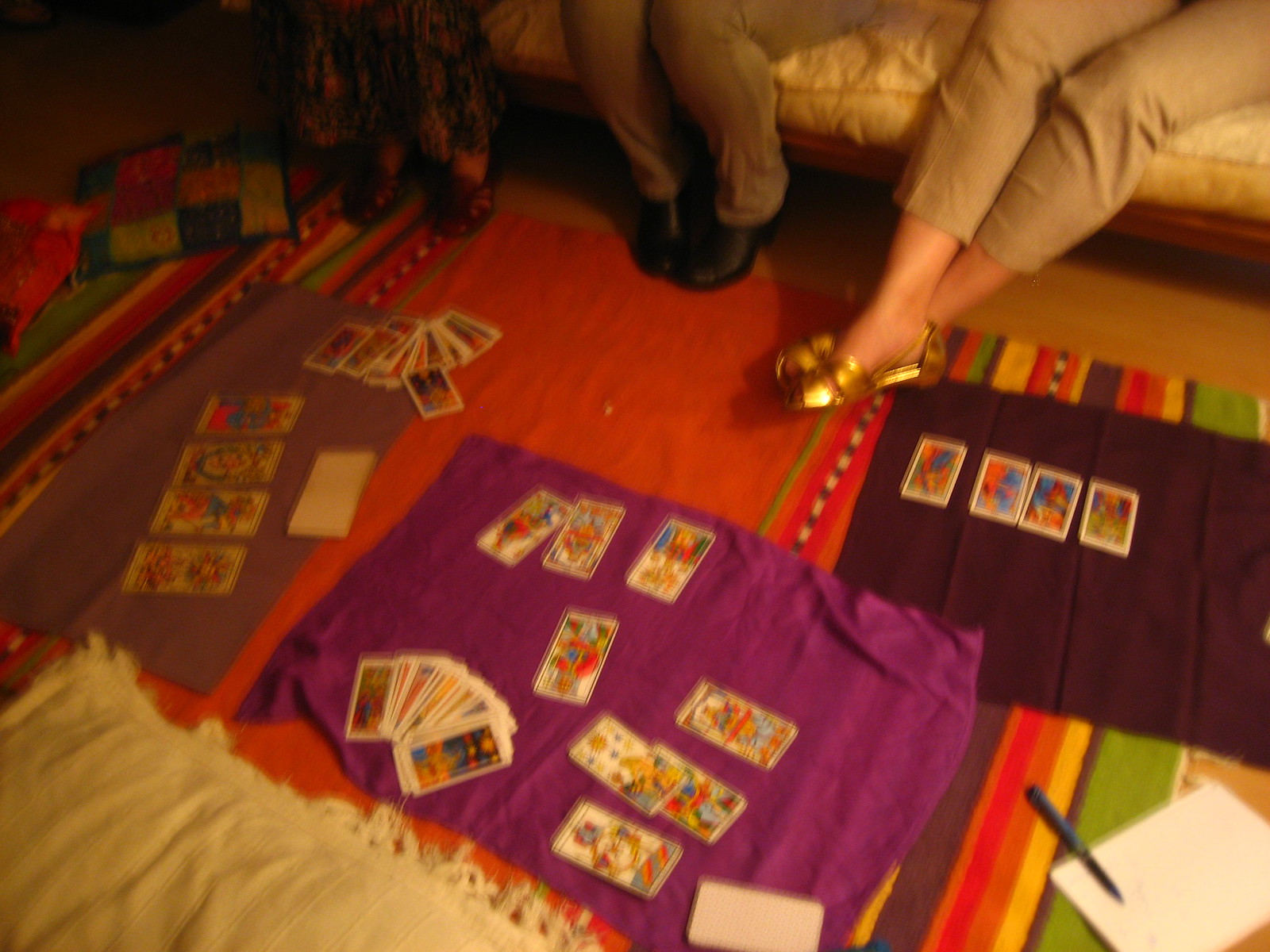The photograph, though slightly blurry, captures a cozy living room scene centered around a cream-colored couch with a wooden frame at the bottom. The upper portion of the image showcases a lineup of three individuals seated on the couch. From left to right, one individual is seen wearing dark-colored pants with brown shoes, the next person sports khaki pants paired with black shoes, and the third individual dons khaki-colored capris and gold shoes. Only their legs are visible in the photograph.

Dominating the foreground is a vibrant orange rug adorned with vertical stripes in varying hues of green, yellow, and brown. Scattered on the floor in front of the rug are multiple layers of additional rugs and various cards. To the upper left, a brown rug features four larger cards, each with distinct pictures, laid at an angle. Adjacent to this, smaller cards are dispersed in a small, spread-out pile.

Further to the right, a purple towel acts as a mat for a spread of diverse cards along with a fan-arranged pile. The top right corner of the image, next to the person with gold shoes, includes a black towel displaying four cards in a neat row. Just above it, a piece of paper and a blue pen complete the intriguing mess, contributing to the detailed and interactive visual tableau.